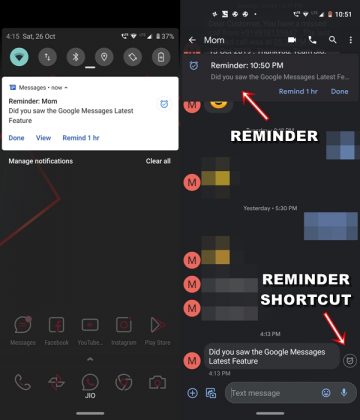A screenshot captures a reminder app on a mobile device with a predominantly black background. At the forefront is a white pop-up screen featuring a reminder titled "Mom." The reminder reads, "Did you see the Google messages latest feature?" Below the text are three clickable options: "Done," "View," and "Remind in One Hour." Adjacent to these options, the screen details the scheduled time for the reminder, which is 10:50 p.m. The app also shows a blurred-out section indicating a text message exchange between the device and "Mom," although the content of the messages remains unreadable.